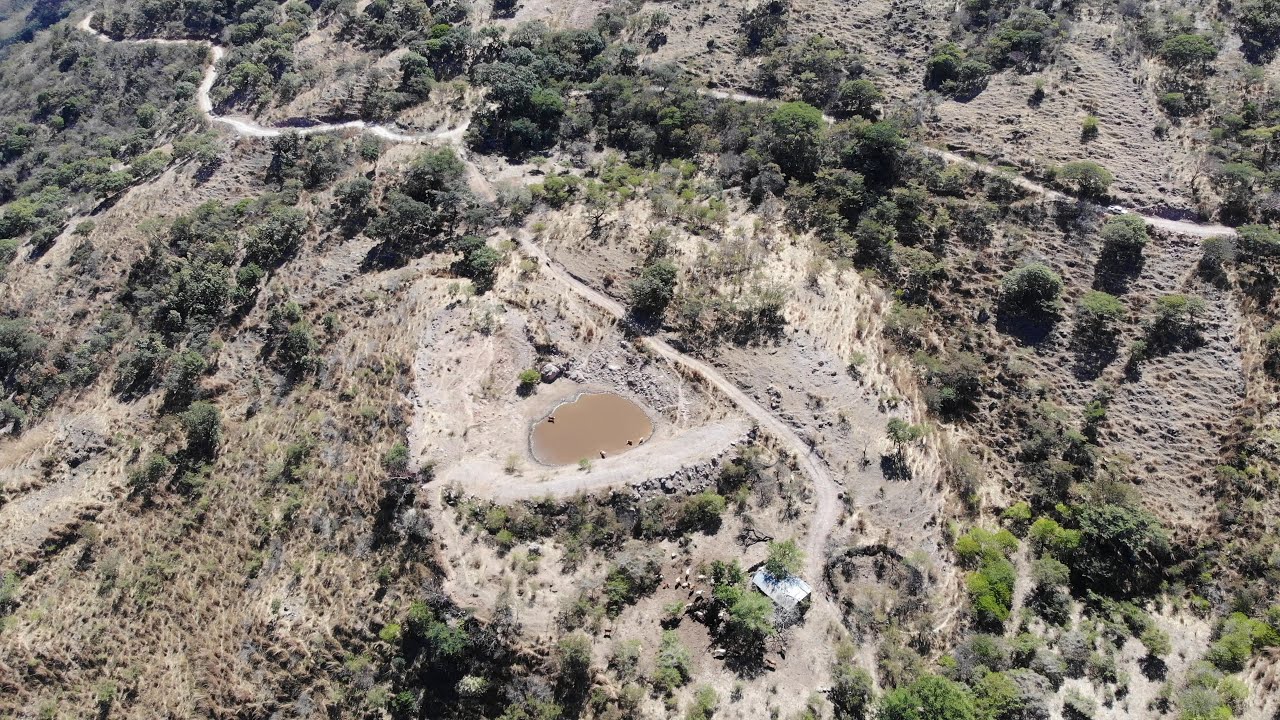The image is a top-down aerial view of a dry, rural landscape with sparse, green trees and patches of bushes dotting the sandy or desolate terrain. At the center lies a dark brown lake or pond, where people can be seen swimming. Adjacent to the pond is a small rectangular building with a metal gray roof, and nearby, there's a circular walled pasture. Three unpaved roads intersect towards the center of the image, forming a network that connects the different elements within the landscape. These roads wind through the scene, with one running diagonally from the bottom right towards the upper left, another stretching horizontally from the right midsection to the left middle, and a connecting path meeting up towards the center. The entire scene is bathed in abundant sunlight, indicating it is taken during the daytime, imparting a dry yet vibrant atmosphere to the photograph.